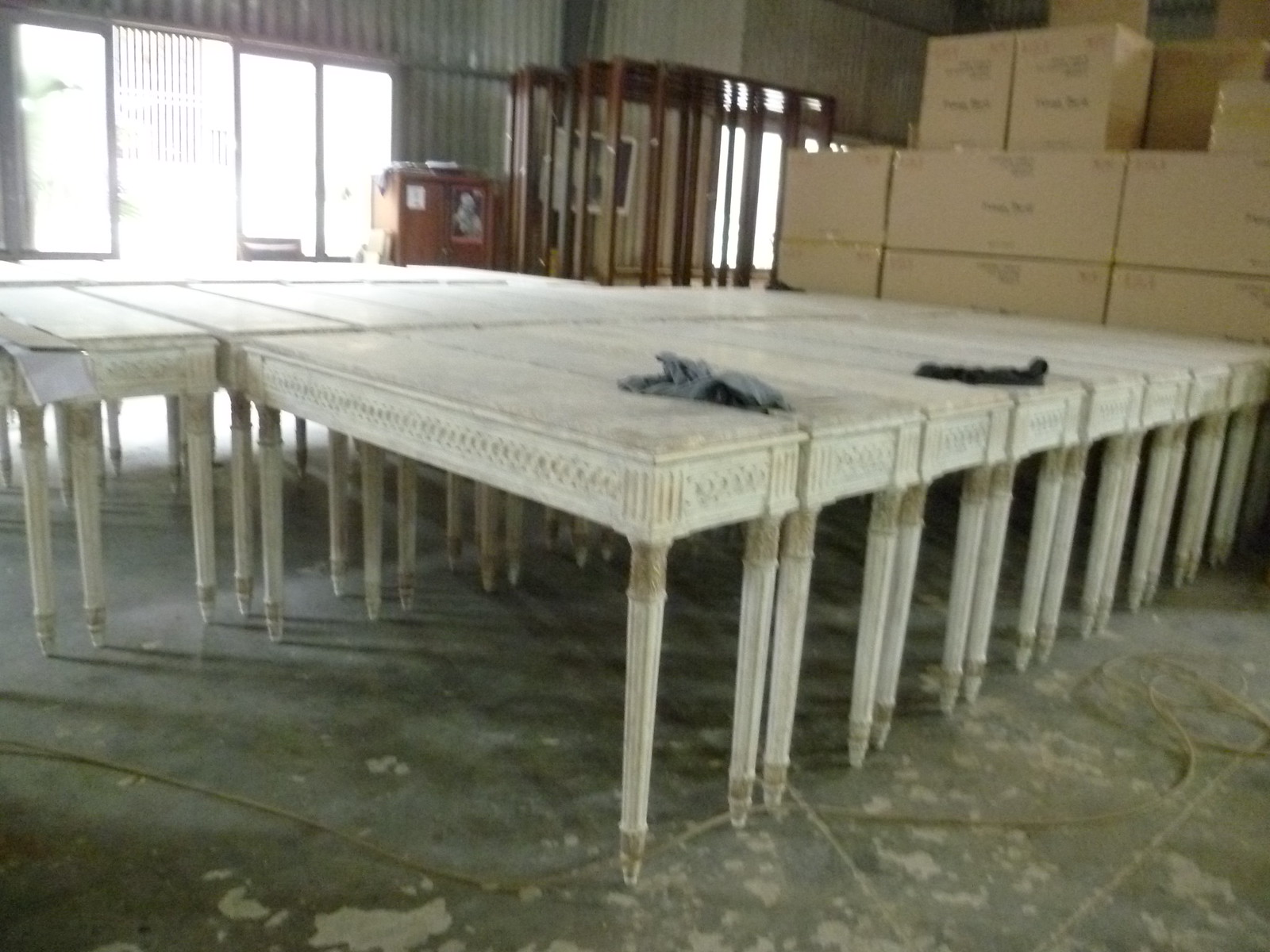This somewhat blurry, soft-focus landscape color photograph portrays what appears to be a warehouse or factory storage area. Dominating the scene are several rows of identical white, ivory-colored console tables, possibly manufactured or stored here. They are neatly lined up in a sequence of rows stretching towards the back left of the image. Each table features a detailed design on the apron, although these areas exhibit signs of wear, appearing dirt-colored. The tables' square legs, which taper to sharp points at the floor, stand on a well-worn, dark green cement floor marred with grey patches from peeling or damage.

To the back right, stacks of cardboard boxes rise high, resembling packing cartons. Sparse details populate the scene, including a pair of work gloves visible on two of the tables and a red cabinet in the background. The cabinet, with what appears to be a statue on its top shelf, is illuminated by natural light streaming in through windows positioned above the tables. The overall impression is one of an aged and functional industrial space, softened by the photograph’s blurred quality.